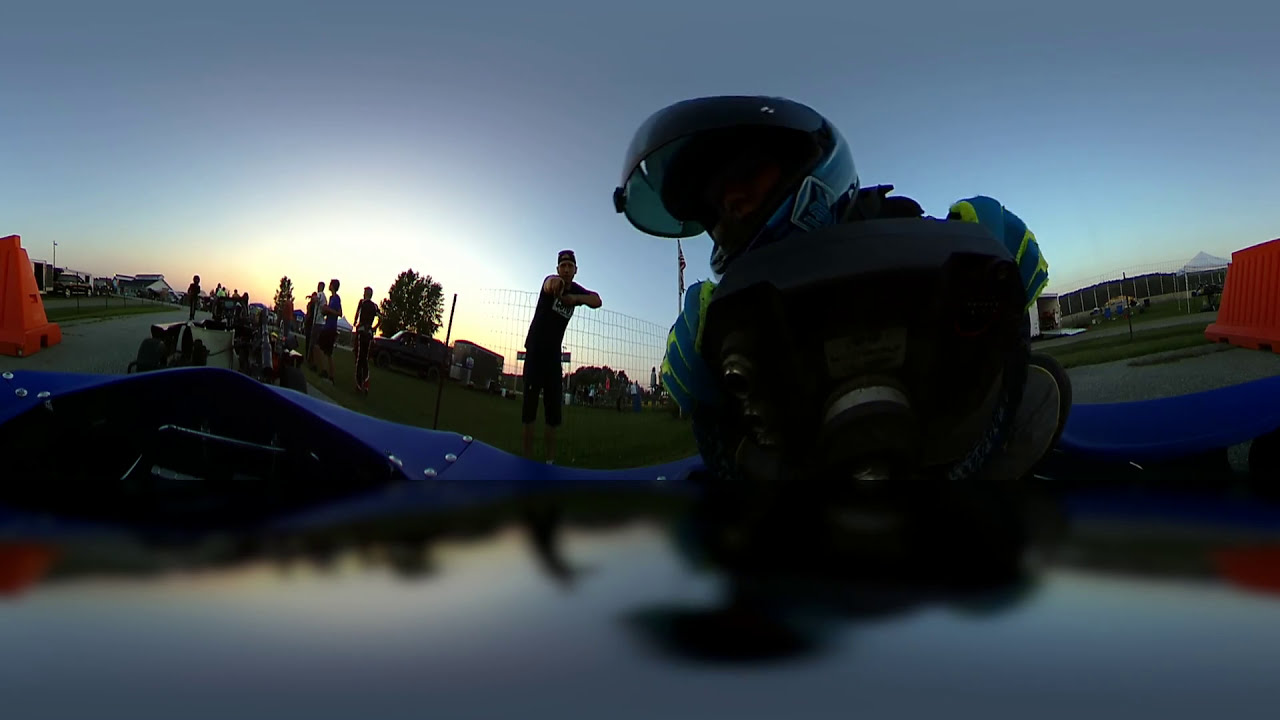The image appears to be distorted, showing a complex outdoor scene during either early morning or late evening with a gradient sky transitioning from light blue to dark gray. In the foreground, there is a reflection on a shiny surface, possibly the hood of a car, and the partial, shadowed view of a person situated on the right side. This person, who might be on a motorcycle or perhaps a go-kart, has their head tilted slightly left, and we can see their helmet or other sports equipment. Below them, there are potentially gloved hands in yellow and green, holding what seems to be handlebars or a steering wheel.

Beneath this setup, there appears to be a wire fence and an orange pylon. Behind the main figure, in the grassy area, stands a man with an arm raised and pointing towards the camera. Additional figures are to the left, shaded and somewhat indistinct. To the right, a small building is visible in the background, along with a road and a few distant houses. A red barrier and a field also feature in this dynamic, multi-faceted outdoor scene.